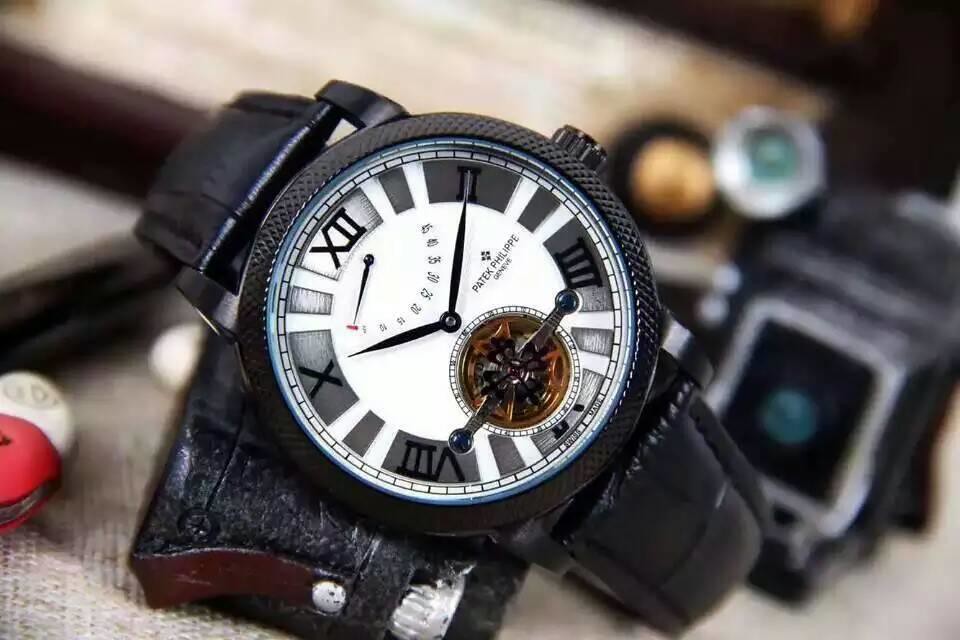This is a highly detailed color photograph that prominently features an elegant wristwatch in sharp focus, dominating the foreground. The focus on the watch is so crisp that it reveals the intricate design elements, while the background remains a blur of indistinct shapes and colors. The wristwatch boasts a sophisticated analog dial with a predominantly white face and is adorned with Roman numerals marking the 12, 2, 4, 6, 8, and 10 positions. The black hour and minute hands are centrally riveted, while a smaller second hand arcs below the "XII" (12) within a semi-circular dial graduated from 5 to 45 in increments of 5. 

The watch is housed in a black metal frame, complementing its black leather strap, which extends around the back and subtly props the watch at a slight angle. This angle requires viewers to tilt their heads 45 degrees anti-clockwise to read the time correctly. Notably, the watch brand, "Patek Philippe," is clearly inscribed along with "Genevieve" just below it. There is also a visible circle at the bottom of the watch face, offering a glimpse into its intricate gears, with two rods ending in small black metal balls.

The composition of the background hints at other objects, their blurred outlines suggesting possibilities like another watch, an old-fashioned camera, and a red tool or pocket watch, although their precise identities remain indistinct. The watch rests on what appears to be a white canvas surface, adding to the textured contrast and overall aesthetic of the photograph.